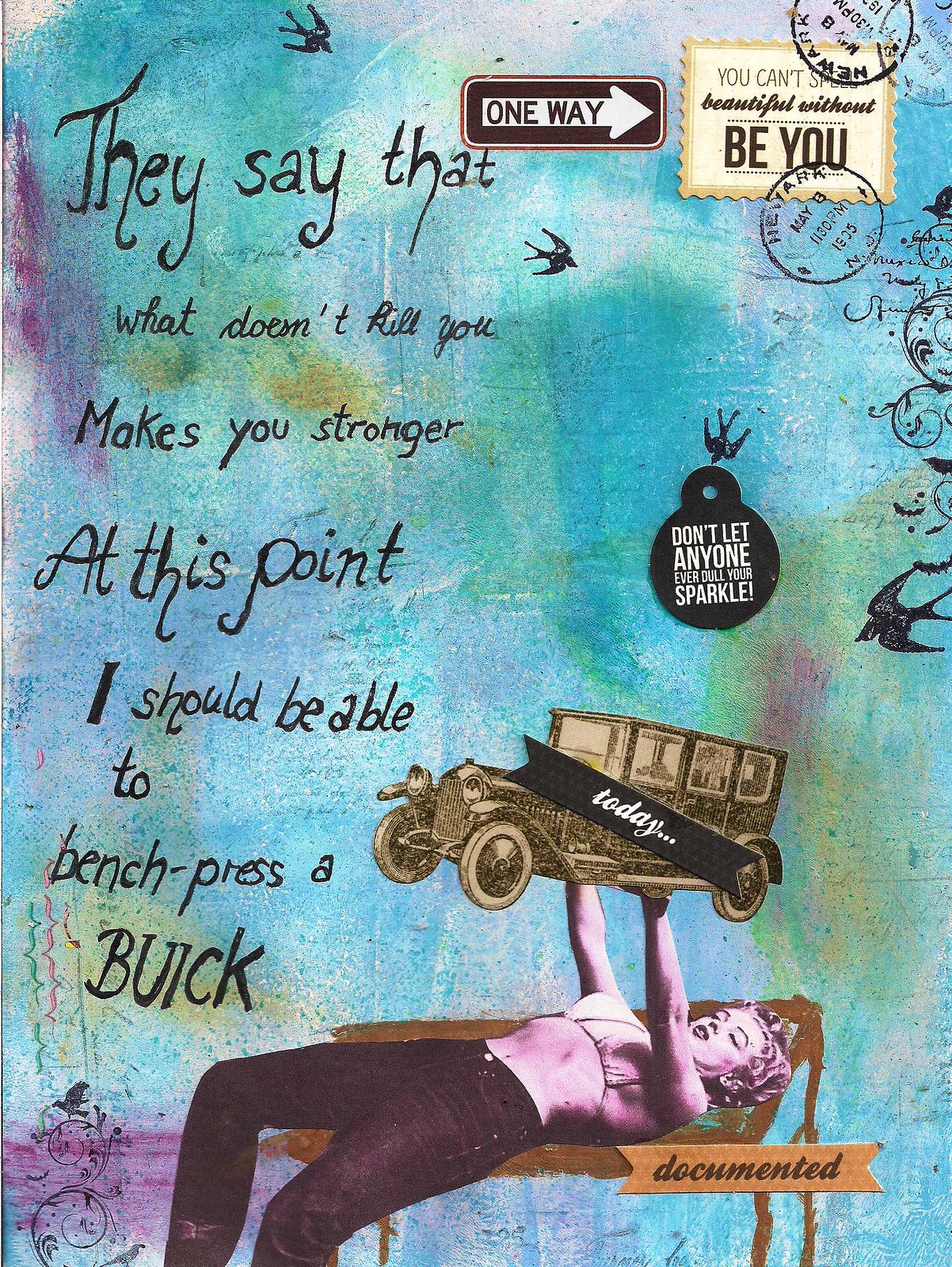This vibrant and playful postcard features a dazzling array of elements that are sure to bring a smile to anyone's face. Set against a whimsical, watercolor-inspired backdrop of baby blue, green, and hints of purple, the image is adorned with charming black bird silhouettes and swirling accents. 

Centered prominently on the left side, a delicate, dainty font spells out the humorous and empowering saying, "They say that what doesn't kill you makes you stronger. At this point, I should be able to bench press a Buick." Complementing this, a blonde woman, with an appearance reminiscent of Marilyn Monroe, is depicted laying on her back with arms extended upwards, effortlessly lifting a brown Buick from the 1930s. Her attire includes jeans, a bare midriff, and a bra, exuding a mix of strength and vintage charm. 

The postcard is sprinkled with various sticker-like icons, including a one-way street sign pointing towards the main stamp, which bears the uplifting message, "You can't be beautiful without being you." Additional stamps scattered across the card mimic those seen on mailed letters, enhancing its nostalgic feel. 

Details such as a banner from the upper portion of the Buick to the back tire with the word "Today" in white letters on black, and another brown banner underneath her arm inscribed with "Dark Prince is documented," add layers of intrigue and depth to the composition.

Overall, this postcard seamlessly blends humor, inspiration, and a touch of retro flair, creating a delightful and memorable piece of art.